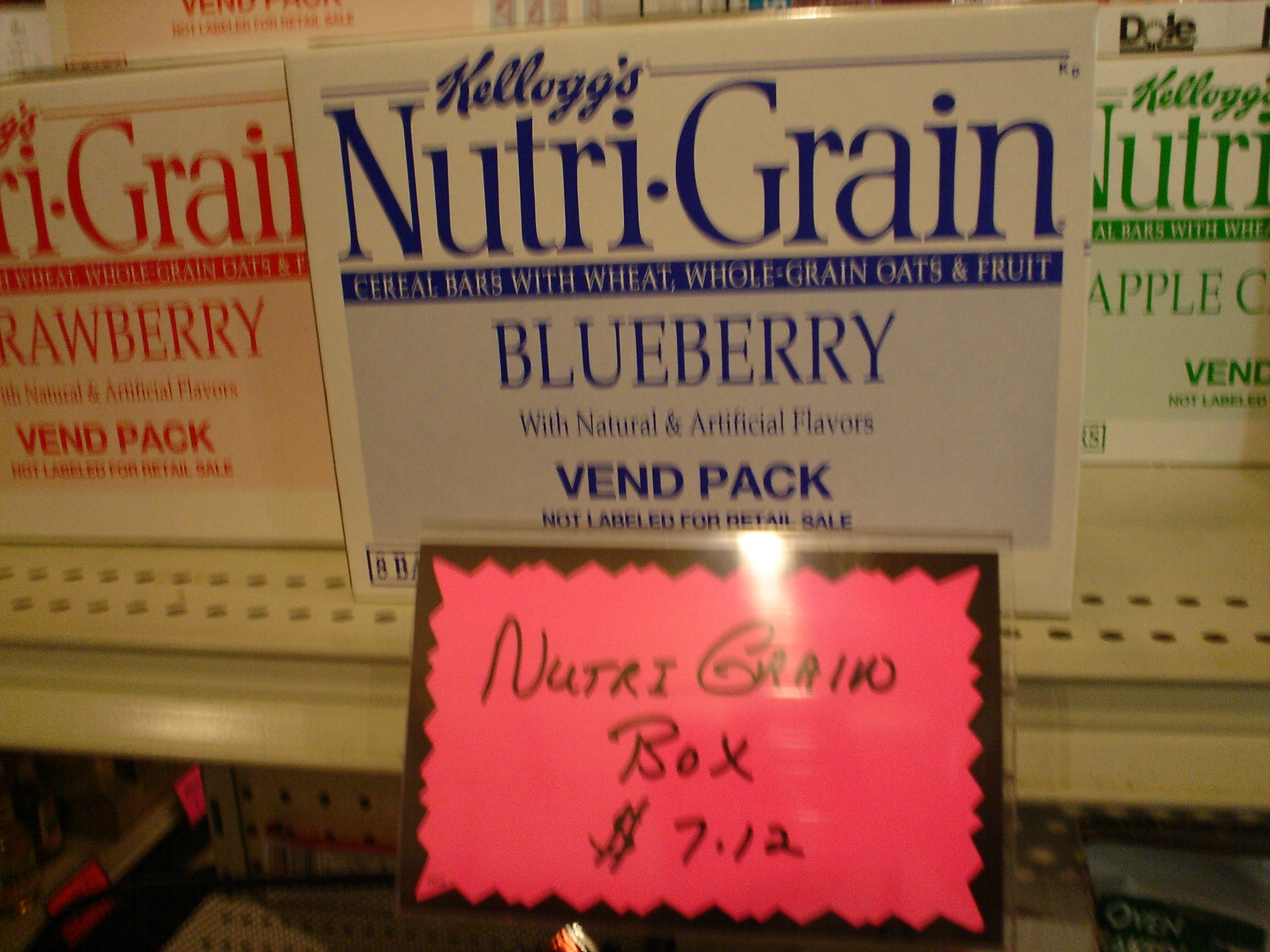This is a photograph of a store shelf displaying Kellogg's Nutri-Grain cereal bars. The shelf highlights various flavors of Nutri-Grain bars in clearly labeled boxes. The central box, prominently featured, is a blueberry variant, characterized by a white box with dark blue lettering. To its left, there's a half-visible box with red lettering, indicating the strawberry flavor. On the right, partially obscured, is a green-labeled box, denoting the apple cinnamon flavor.

Each box shares a consistent design: the Kellogg's logo at the top left corner, followed by the large Nutri-Grain brand name, and an orange banner stating, "cereal bars with wheat, whole grain, oats, and fruit." Underneath, the respective flavor (Strawberry, Blueberry, Apple Cinnamon) is highlighted in bold letters, with notices regarding natural and artificial flavors, and a label indicating "VendPak, not labeled for retail sale."

Below the Nutri-Grain boxes on the shelf, a laminated poster adhered to a metallic shelf bracket features a hot pink tag with a black border, displaying the price "$7.12" for the box of Nutri-Grain bars in black handwriting. Below this front shelf, additional shelving is visible, but the items are cut off in the photograph. The blurred nature of the image adds an element of presumed convenience store ambiance, focusing on the sale of full Nutri-Grain boxes rather than individual bars.